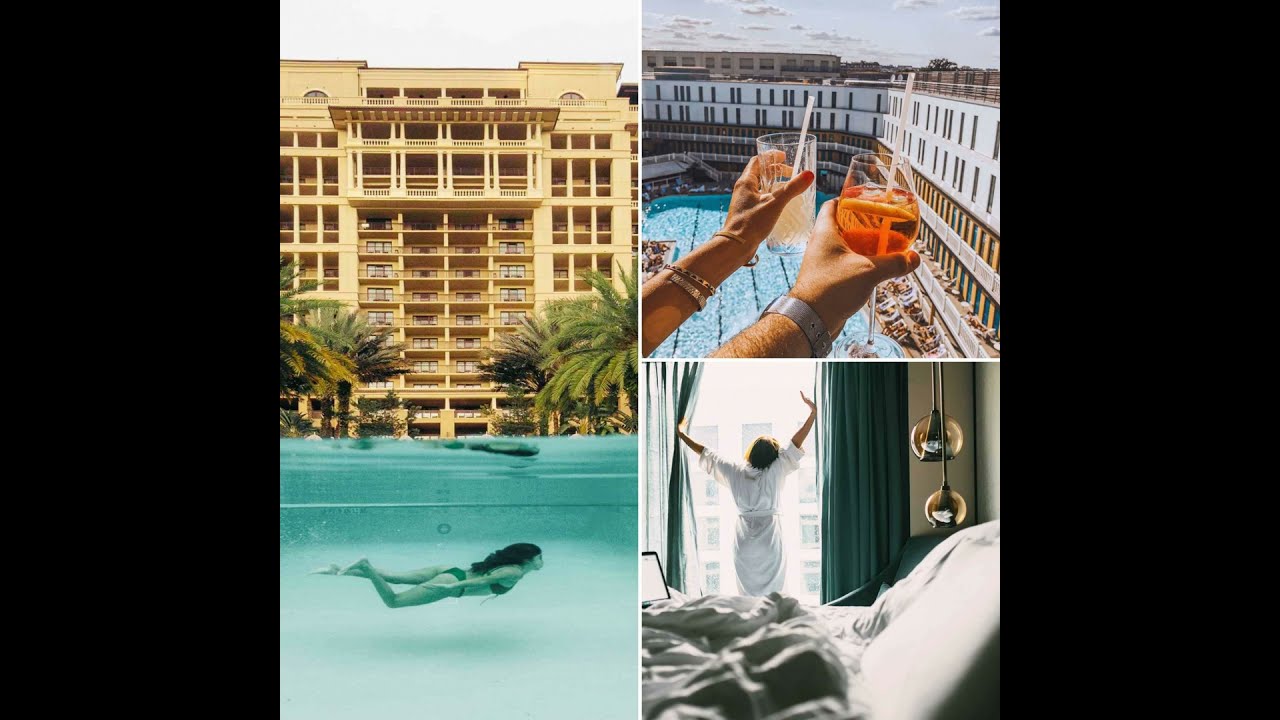A horizontal photo collage composed of three distinct yet connected images. On the left, a vertical image showcases a tan-colored, multi-story hotel with palm trees in front of it. In the foreground's bottom, a woman can be seen swimming underwater in a clear blue pool. To the right, the collage is divided into two smaller, equal-sized rectangles. The top right section highlights a close-up of a woman's and a man's hands holding glasses filled with drinks, as if making a toast. They stand on a balcony overlooking a large pool and the surrounding hotel building, giving a sense of relaxation and celebration. Below this, the bottom right image depicts a woman in a white robe stretching with her back to us, standing in front of a tall window with green curtains. Morning light floods the room, illuminating a messy bed with scattered pillows and a blanket. The overall composition conveys an atmosphere of luxury, leisure, and the serene moments of a morning at an upscale resort.